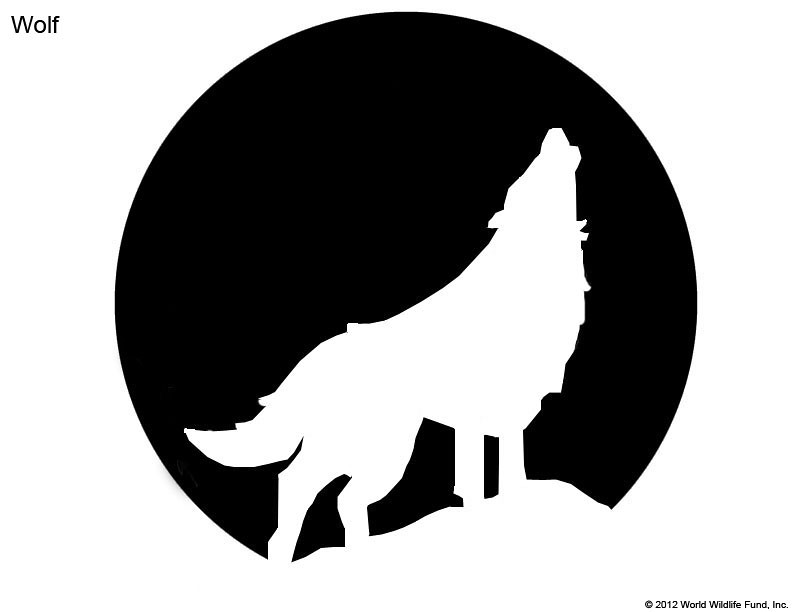This image features a minimalistic and iconic logo with a stark black and white color scheme. At the center, encased in a black circle, is the white silhouette of a cartoon-like wolf standing on a jagged cliff, howling upwards towards what would typically be the moon, but in this design, the moon is represented by the black background, creating an inverse effect. The use of contrasting colors creatively highlights the howling wolf and the cliff.

In the top left corner of the image, outside the black circle, the word "Wolf" is inscribed in a near Arial font in black text. In the bottom right-hand corner, there is a copyright symbol, ©, followed by "2012 World Wildlife Fund, Incorporated," in black. This elegant design evokes a sense of wilderness and the night, and could serve as a logo or an artistic representation for the World Wildlife Fund.